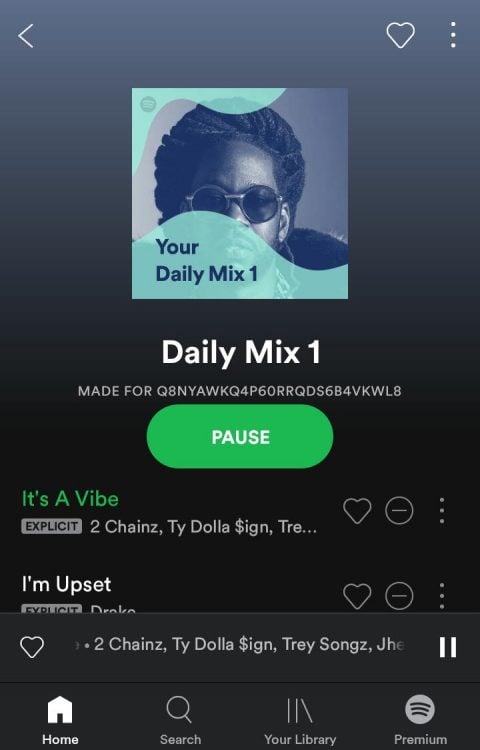**Caption:**

A mobile screenshot showcasing Spotify's "Daily Mix 1" playlist interface. The screen features a dark background with various elements arranged strategically:

- **Top Left:** An arrow pointing back to the previous screen.
- **Top Right:** A comically styled Valentine's heart icon followed by a three-dot menu.
- **Upper Section:** The iconic Spotify logo accompanied by an avatar portraying a black man with large black sunglasses and voluminous black hair.
- **Bottom Left Corner:** A wavy line in white and light green colors.
- **Bottom Right:** The text "Your Daily Mix 1" in white, with subtext reading "Daily Mix 1". Below this, in gray, it says "Made for" followed by an extensive string of alphanumeric characters.
- **Center:** A green play/pause button with the label "Pause" in white.
- **Left Side:** The phrase "It's a vibe" in green text, with "Explicit" and the names "2 Chainz, Ty Dolla $ign, and Trey" listed in gray beneath it.
- **Right Side:** Another occurrence of the heart icon, a circle with a line through it, and the three-dot menu. Beneath these, the text "I'm Upset" in white, with "Explicit" and the barely readable name "Drake".
- **Bottom Right:** Again, the heart icon, the text "Plus 2 Chainz, Ty Dolla $ign, and Trey" indicating the song currently playing.
- **Bottom Section:** A row of icons:
  - A house icon labeled "Home".
  - A gray magnifying glass labeled "Search".
  - An icon depicting two horizontal lines stacked vertically labeled "Your Library".
  - The Spotify logo accompanied by the word "Premium".

This detailed description captures every element visible on the screen, providing a comprehensive understanding of the Spotify mobile interface.